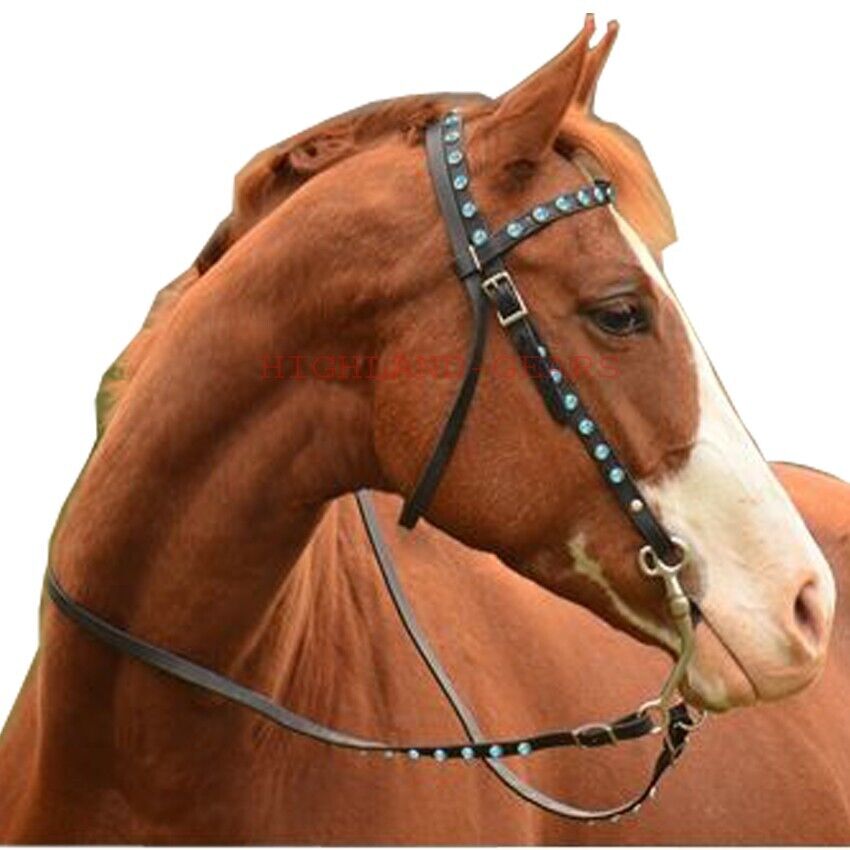This detailed photograph showcases a close-up of a horse against a white background, indicating it has likely been digitally edited or placed onto the background as suggested by the slightly pixelated outlines. The horse is captured in a profile view, turning its head so it gazes down to the right side. Its neck is bent diagonally, presenting a striking and attentive pose with perked up ears. The horse's coat is a beautiful ginger or chestnut brown color with a matching mane. A distinctive white patch runs from the center of its forehead down to its white muzzle. The horse is adorned with a black leather bridle that is embellished with silver-blue studs or rhinestones, providing an ornate detail to the image. Notably, the horse's eyelashes are beautifully visible, adding to the elegance of the portrait. There is a barely noticeable text blending with the horse which begins with "H-I-G-H," though the rest of the letters are difficult to discern.